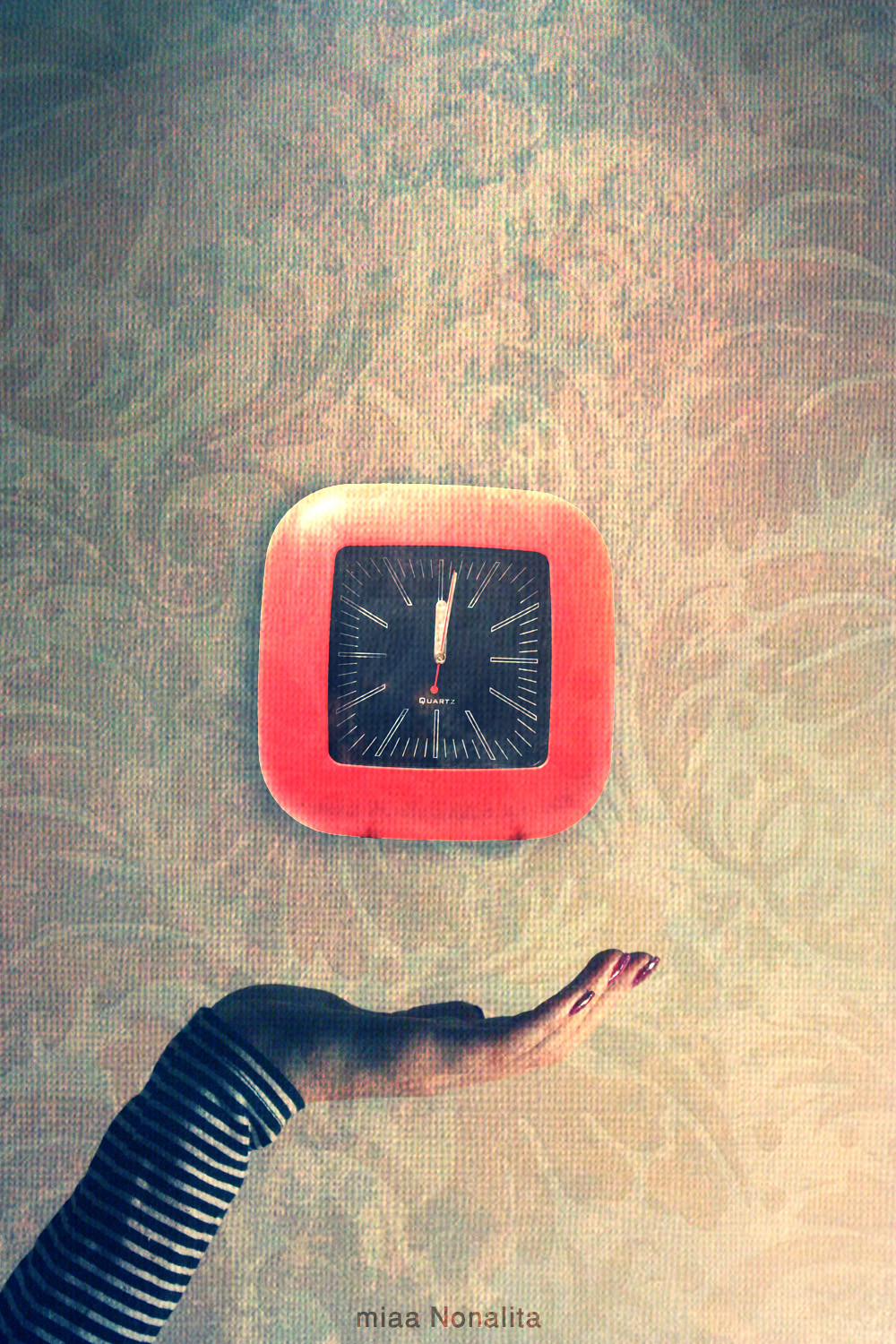The image depicts an artistically photographed scene featuring a detailed and textured background resembling old-fashioned, pastel floral wallpaper with muted pinks, greens, blues, and whites. The wallpaper's brightness varies, being more vivid at the top and sides and gradually fading towards the center and lower right. Centrally positioned on the wall is a square clock with rounded corners, bordered by a prominent red frame. The clock face, encased within a black inner square with rounded corners, has no numbers, only white dashes and hands. The hour and minute hands point upwards, while a red second hand indicates five minutes past twelve. Below the clock, a woman's hand, palm facing up and adorned with dark red nail polish, appears to cradle the clock without touching it. The forearm is clad in a blue and white striped long-sleeved shirt. Below this scene, text reads "M-I-A-A" followed by "N-O-N-A-L-I-T-A."